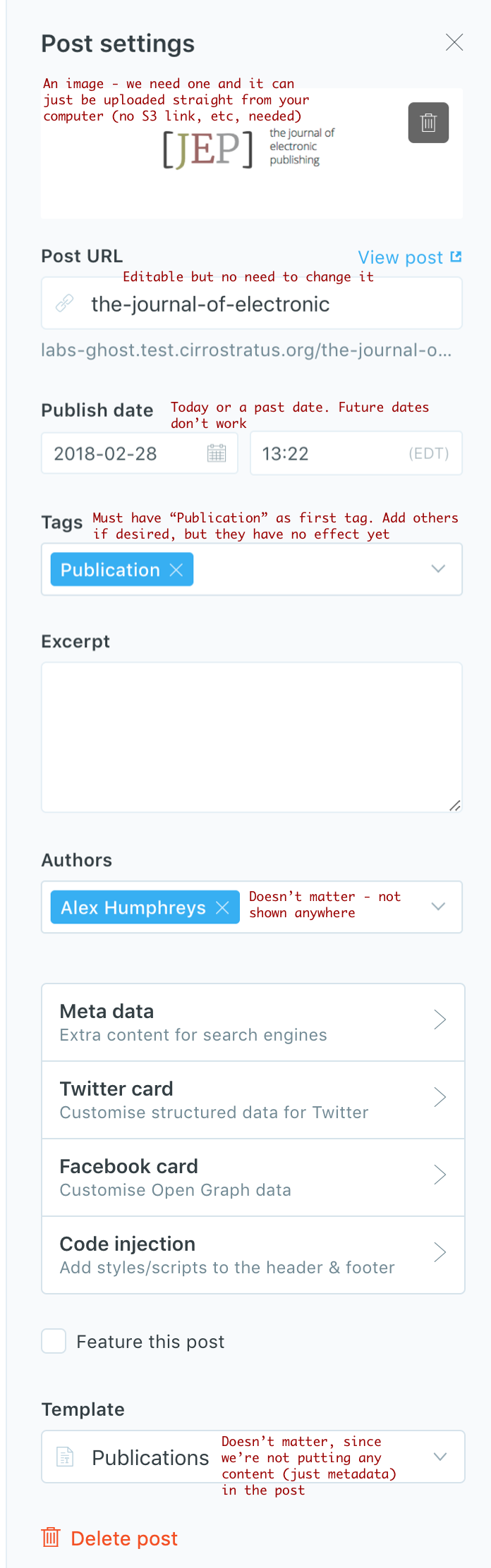The image displays the post settings interface of a content management system, featuring various options and fields for configuring electronic publications. The background is a neutral gray, providing a clear view of the elements present on the screen.

The main focus is a rectangular section possibly representing a trash can icon. The interface includes important functionalities:
1. **Post URL**: A text field to input the URL where the post will be accessible; it shows a sample URL "thejournal-electroniclab-goes.test.status.org/thejournal-row...".
2. **Date Settings**: Options to choose publication dates, although only past and present dates are functional.
3. **Time Picker**: Displaying "13:22 ADT" set for the publication on the 28th calendar day.
4. **Tags Section**: Required to include "publication" as the first tag followed by optional tags that hold no influence yet. 
5. **Author Information**: Displays a black text name, "Alex Humphreys," highlighted in a blue rectangle.
6. **Metadata Section**: Allows for additional searchable content to be added, featuring dropdown menus and text fields.
7. **Social Media Cards**: Settings for customizing data shown on Twitter and Facebook.
8. **Code Injection**: Offers the ability to add extra script or style code to the post header.
9. **Post Template Options**: Contains settings related to the publication template, marked as irrelevant in this context.
10. **Trash Can Icon and Delete Post**: Red text referencing the option to delete the post.

The caption neatly consolidates various configurations and the interface’s look, emphasizing that electronic publishing is turned off.